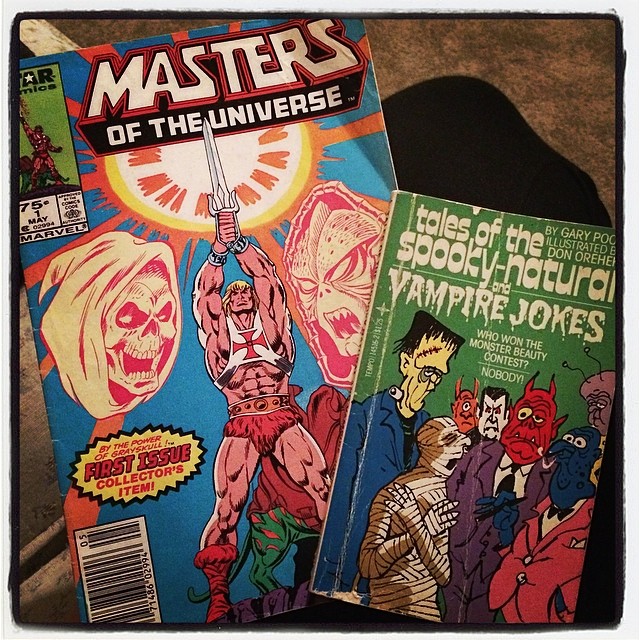In the image, two vintage comic books are spread out on a tan surface, possibly near a black mouse pad, against a dark and light brown shaded background. The larger comic book, occupying most of the space, is titled "Masters of the Universe." It features a prominently bulked-up He-Man holding aloft his power sword beneath a bright sun. Flanking He-Man on the cover are two of his foes, with Skeletor on the left and another hooded creature on the right. There is a yellow starburst outlined in black and red letters that proclaims, "By the Power of Grayskull," along with a blurb identifying it as a "First Issue Collector's Item." 

On top of the "Masters of the Universe" comic lies a smaller book titled "Tales of the Spooky Natural and Vampire Jokes" by Gary Pak, with illustrations by Don Orhen, although part of the text is cut off. This comic features cartoonish depictions of a mummy, Frankenstein, a devil, a vampire, and several other ghoul-like characters, all appearing more grim and melancholy than frightening. An example joke pictured reads, "Who won the Monster Beauty Contest?" with the punchline "Nobody" underneath. The overall mood suggested by the characters’ expressions aligns with the book's humorously dark theme.